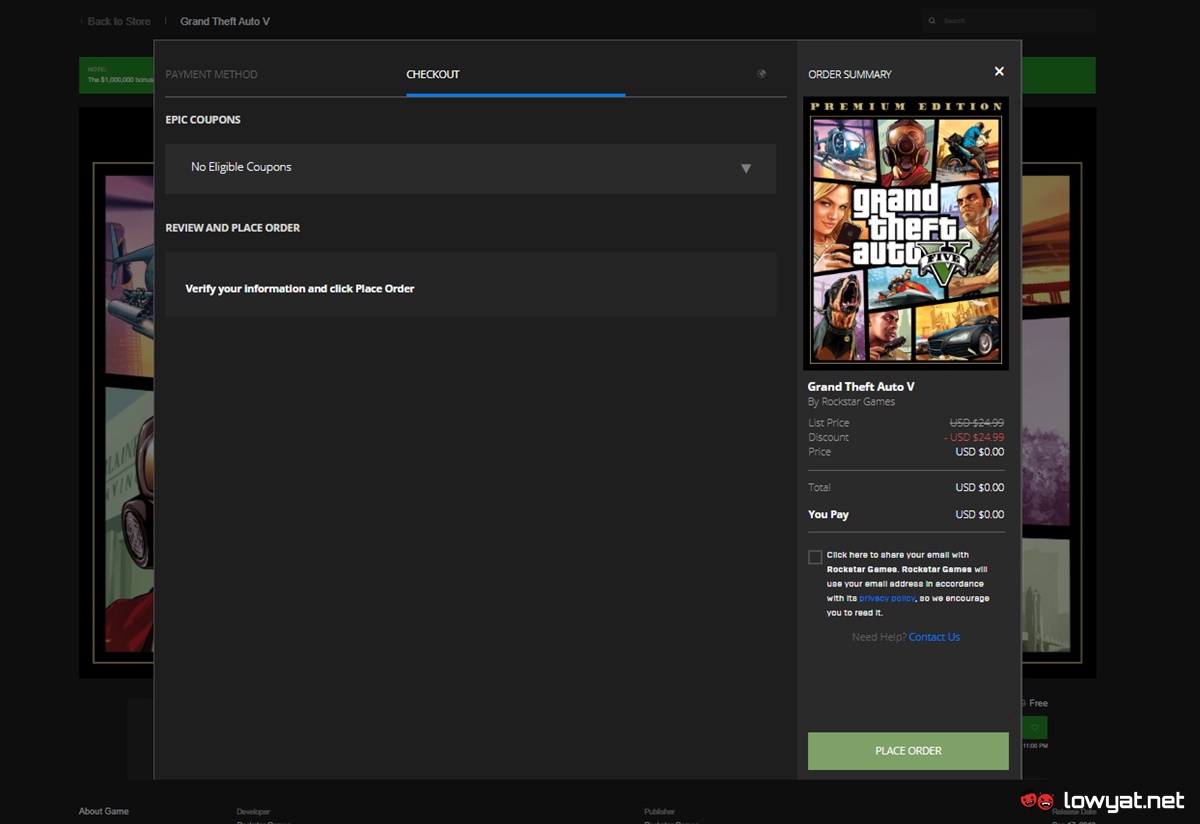This image is a detailed screenshot from a computer screen featuring a checkout process on a website. In the bottom right-hand corner, there's a visible logo that reads "lowyat.net." The background contains various images, partly obscured by a prominent pop-up screen displaying the payment and checkout interface.

The pop-up screen is primarily focused on a checkout section, where "Checkout" is highlighted. Below this, the screen indicates "Epic Coupons" with a message stating "No eligible coupons," accompanied by a drop-down menu for potential coupon selection. Further down, there are instructions to "Review and Place Order" and a prompt to "Verify your information and click Place Order."

On the right side of this pop-up, there is an "Order Summary" section featuring details about a Grand Theft Auto V purchase. An image of the video game's cover is displayed, alongside the title "Grand Theft Auto V by Rockstar Games." The pricing details are broken down as follows: List price - $24.99, Discount - $24.99, resulting in a Price Due of $0. Consequently, the Total amount to be paid is also $0.

There is a checkbox option that reads, "Click here to share your email with Rockstar Games," with a note that Rockstar Games will use the email in accordance with their privacy policy, which they encourage users to read. Additionally, a "Contact Us" link is present for further assistance.

At the very bottom of the pop-up, a large green button labeled "Place Order" is prominently displayed, inviting the user to complete the purchase.